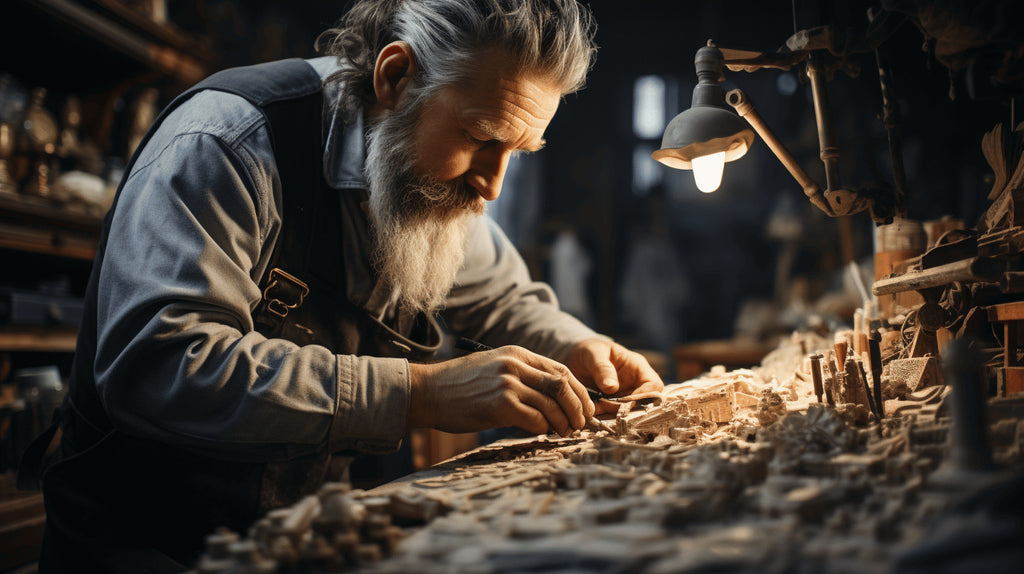In this photograph, an elderly man with long, graying hair and a full gray beard is depicted meticulously working in a dimly lit workshop. He is seated at a cluttered desk, illuminated by a prominent black work lamp with a white bulb and gold accents. The man is dressed in a long-sleeved denim shirt, black suspenders, and a leather apron, suggesting he is engaged in detailed craftsmanship, likely involving wood. The desk is strewn with numerous intricate pieces and trinkets, hinting at a complex assembly process. He holds a tool or pencil, concentrating on his meticulous work. In the background, a blurred window and shelves laden with indistinct objects provide a sense of depth and context to the setting, highlighting the tranquil ambiance of the workshop.